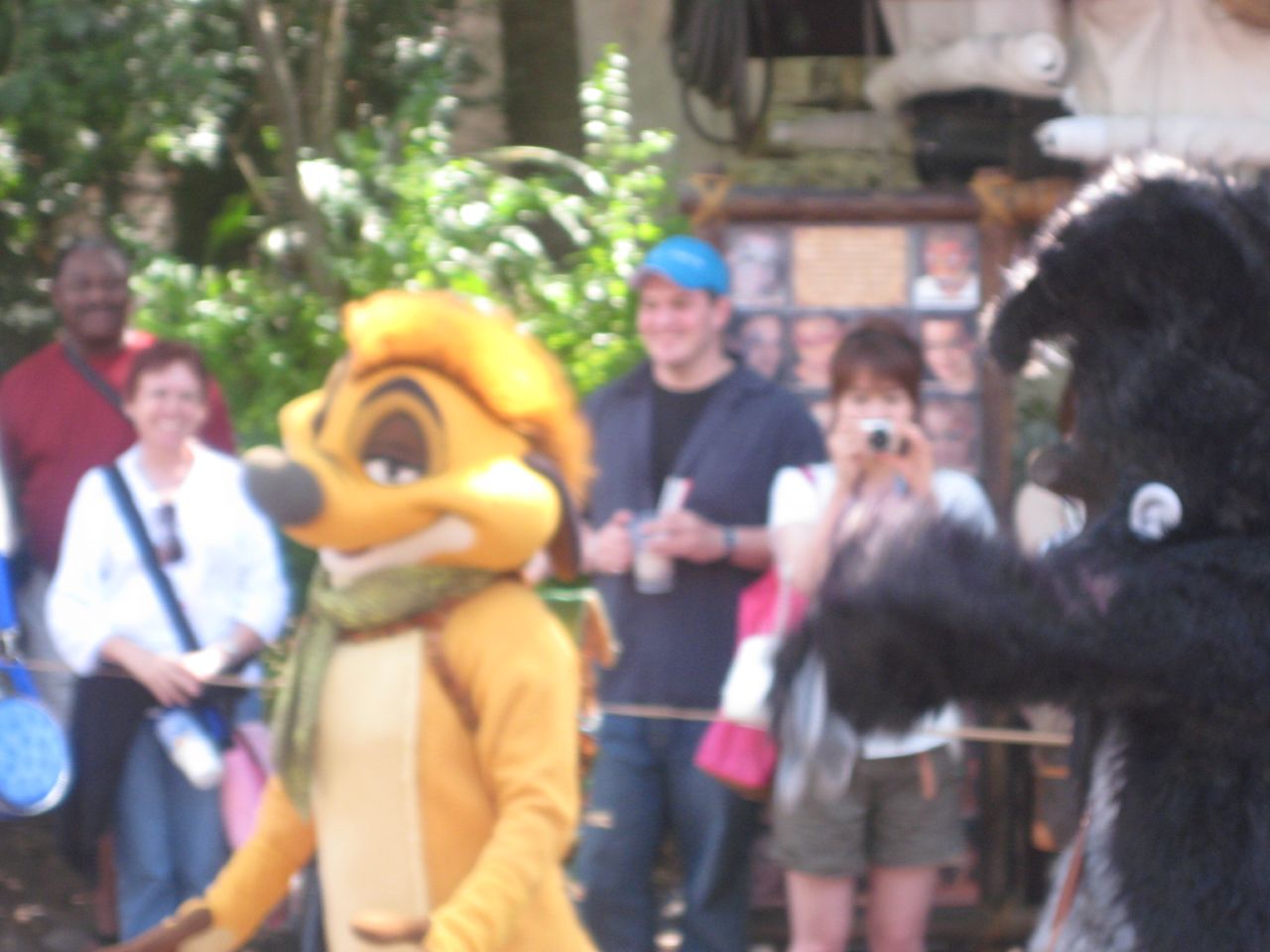In this blurry outdoor photograph, presumably taken at Disney World, we see a character in a Timon costume from "The Lion King," positioned just left of center and facing left. Timon, characterized by his light and dark brown fur, big black nose, large eyes, and distinctive markings, is a clear focal point. On the right-hand side of the frame, partially cut off, is another individual in a black bear costume, as they approach the scene. Behind the characters, a rope barrier prevents the crowd from getting closer; among this crowd is an Asian woman with a camera, capturing the moment. Additionally, other distinguishable figures in the background include a black male in a red top, a white female in a white long-sleeve top, another white male wearing a black top and blue cap, all of whom are smiling and enjoying the scene. The setting is also framed by trees and branches that add to the outdoor ambiance of the moment at this lively, magical gathering.